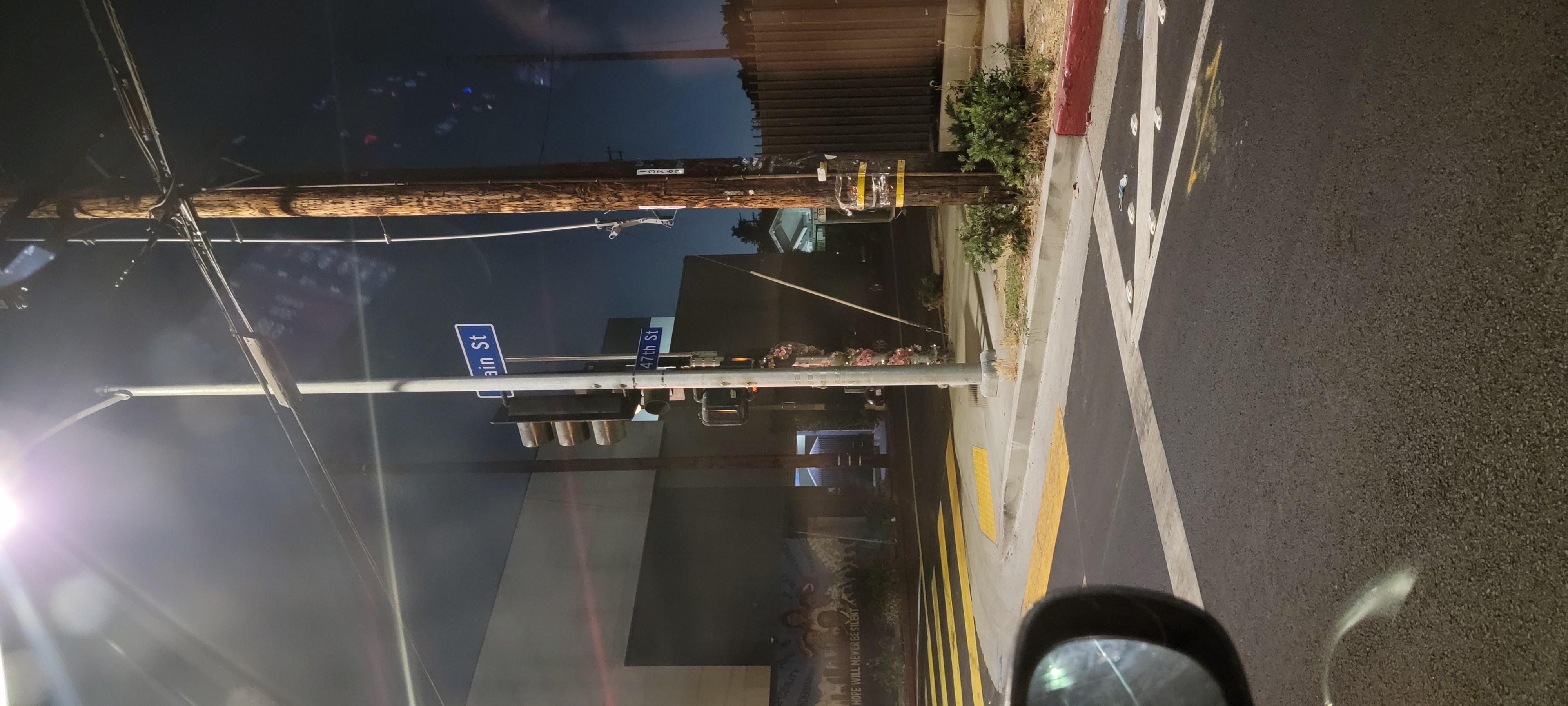This nighttime photograph, rotated a quarter turn to the left, captures a quiet urban intersection from the viewpoint of a vehicle. The scene is illuminated by streetlights, highlighting the dark sky and giving a glimpse of the empty roadway. Prominently visible in the lower part of the image is the car's passenger-side mirror, suggesting the photo is taken from the driver's seat.

The intersection appears to be a four-way crossing, with blue street signs mounted on metal poles marking the corners. Tall streetlight poles stand like sentinels, their lights casting a halo over the asphalt. Adjacent to one of these poles is a telephone pole with power lines extending into the frame, adding to the intricate network of urban infrastructure.

The car is stationed at a pedestrian crosswalk, delineated by distinct white lines on the road. The intersecting street also features a well-marked yellow crosswalk. In the background, a flat-roofed building adds to the cityscape, its silhouette blending into the night.

The street itself is paved with black asphalt, typical of city roads. The curb is marked with a section of red paint, indicating a no-parking or no-stopping zone. At the base of the telephone pole, a small green bush provides a touch of nature amidst the urban environment.